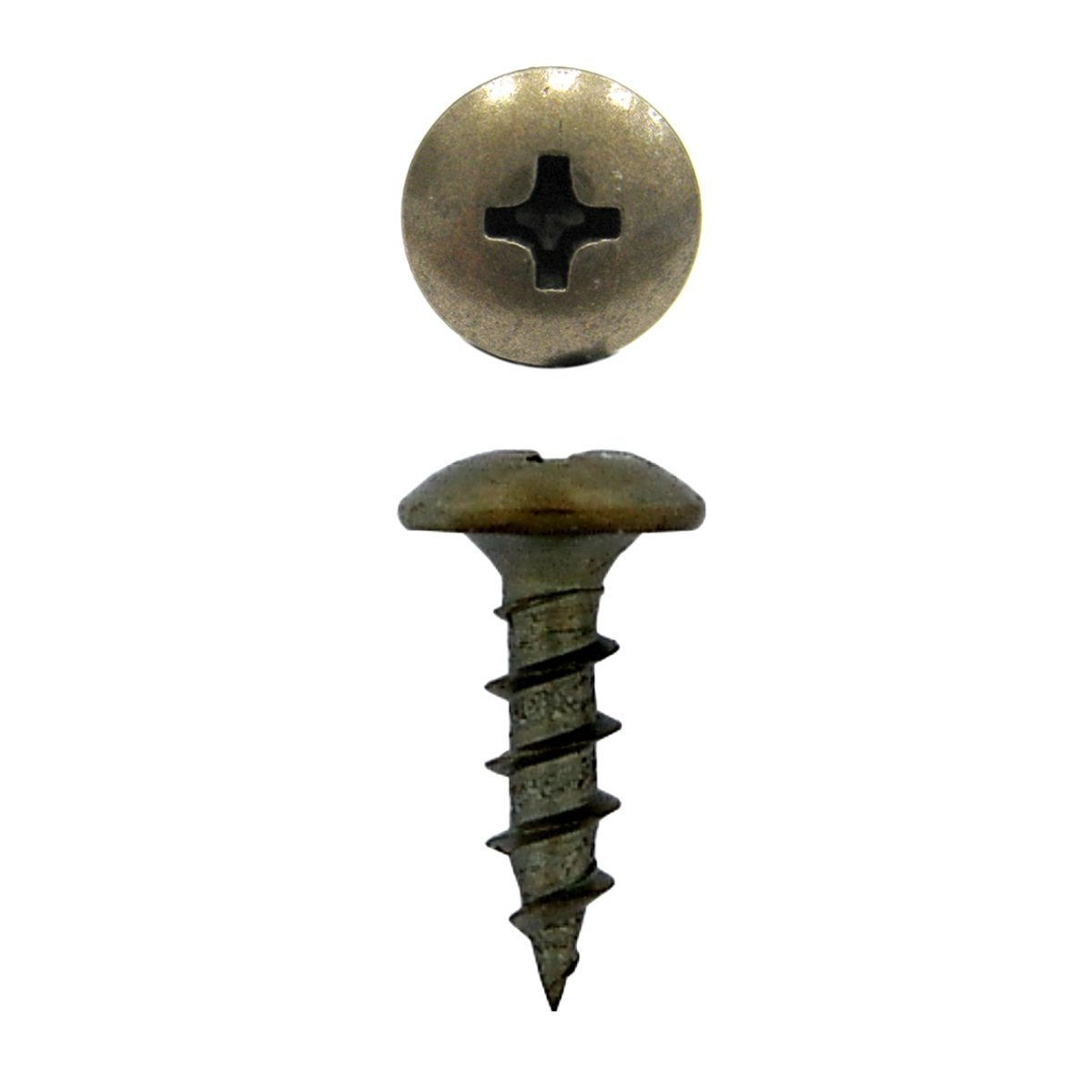The image features two close-up, high-definition views of the same brass-colored, aged wood screw. Set against a stark white background, the top portion of the image displays a view from above, highlighting the screw's round, domed head with a Phillips, cross-shaped indentation. The bottom portion presents a side view, revealing the screw's greenish-brown threading that coils down to a sharp point. The screw's surface shows signs of age with rusty, tarnished edges, yet retains a slight shine and reflections of light on the top third of the head, emphasizing the screw’s timeworn character.